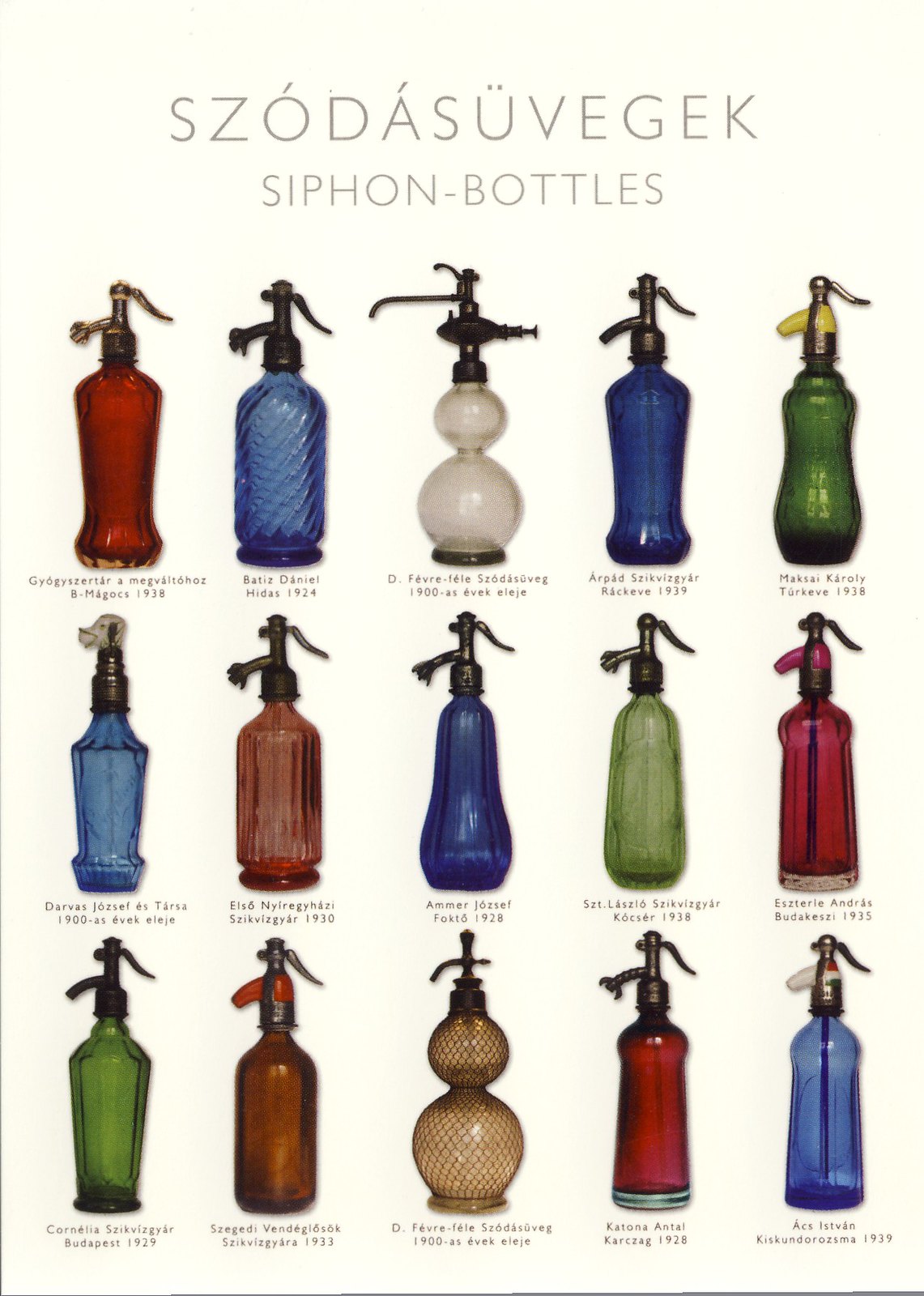The image showcases 15 colorful, vintage siphon bottles arranged in a portrait orientation, with three rows of five bottles each. At the top of the image, in capital letters with accent marks, it reads S-Z-O-D-A-S-U-V-E-G-E-K. Directly below that, in smaller centered text, it says "siphon bottles." Each bottle varies in shape and features a pump top with a bronze appearance. The top row consists of a red bottle, a blue one, a white one, followed by another blue, and a green bottle. In the middle row, the bottles are blue, red, blue, green, and red respectively. The bottom row displays green, red, brown, red, and blue bottles. Beneath each bottle is faint black text, presumed to be dates or years, but it's too small to read clearly. The image is framed with a thin blue line on the left and at the bottom.